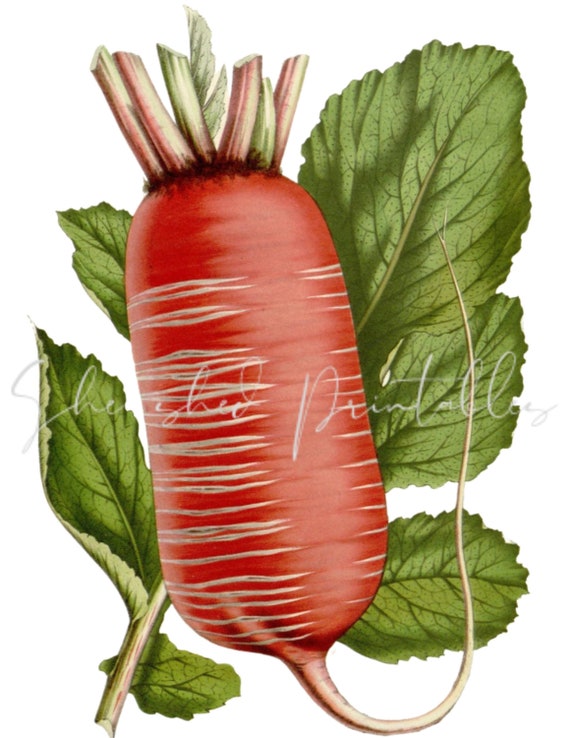This detailed artwork depicts a hand-drawn, long, and fat radish, rendered in ink and watercolor. The radish takes center stage, displaying a reddish-orange hue with brown or white striping along its length. At the bottom of the radish, there is a thin, white root that gradually tapers and curls back up towards the right side. Surrounding the radish, there is a mix of stems and leaves. The upper parts of the stems remain with only small stubs visible, colored in green and red hues, while the background features larger, curling leaves. These leaves have different green intensities, with lighter green undersides and darker green vein patterns in shaded regions. The leaves start smaller towards the bottom left of the image and become significantly larger towards the top right. The entire composition is set against a white background, which slightly obscures some fine, handwritten text—likely the artist’s signature.